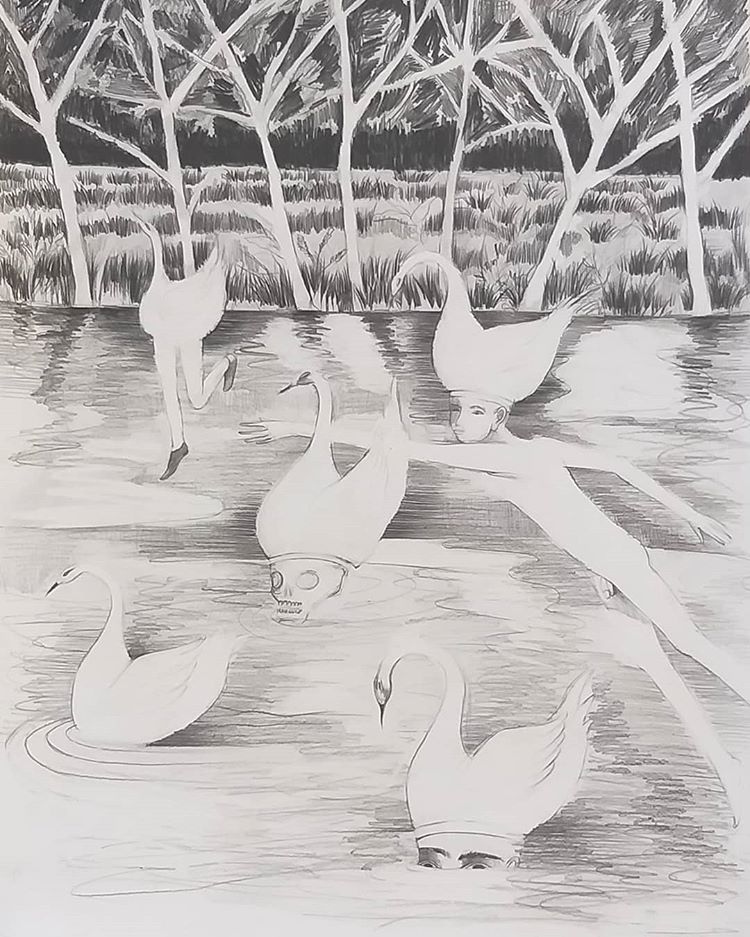This intricate black and white vertical stencil drawing creates an eerie and surreal tableau of a river or lake scene. Dominating the composition, three swans glide across the water, each uniquely transformed. The swan on the left boasts human legs wearing shoes, running over the water's surface. In the middle, another swan reveals a human skull just beneath it, lending a macabre touch. The swan on the right is perched atop a naked boy, whose body is visible just beneath the water, as though the swan is his hat. The detailed pencil etchings capture striking light reflections on the water, against a backdrop of dark skies, tall bundles of grass, and a line of trees with prominent white branches. The trees' reflections shimmer on the water, enhancing the scene's depth and mystery.